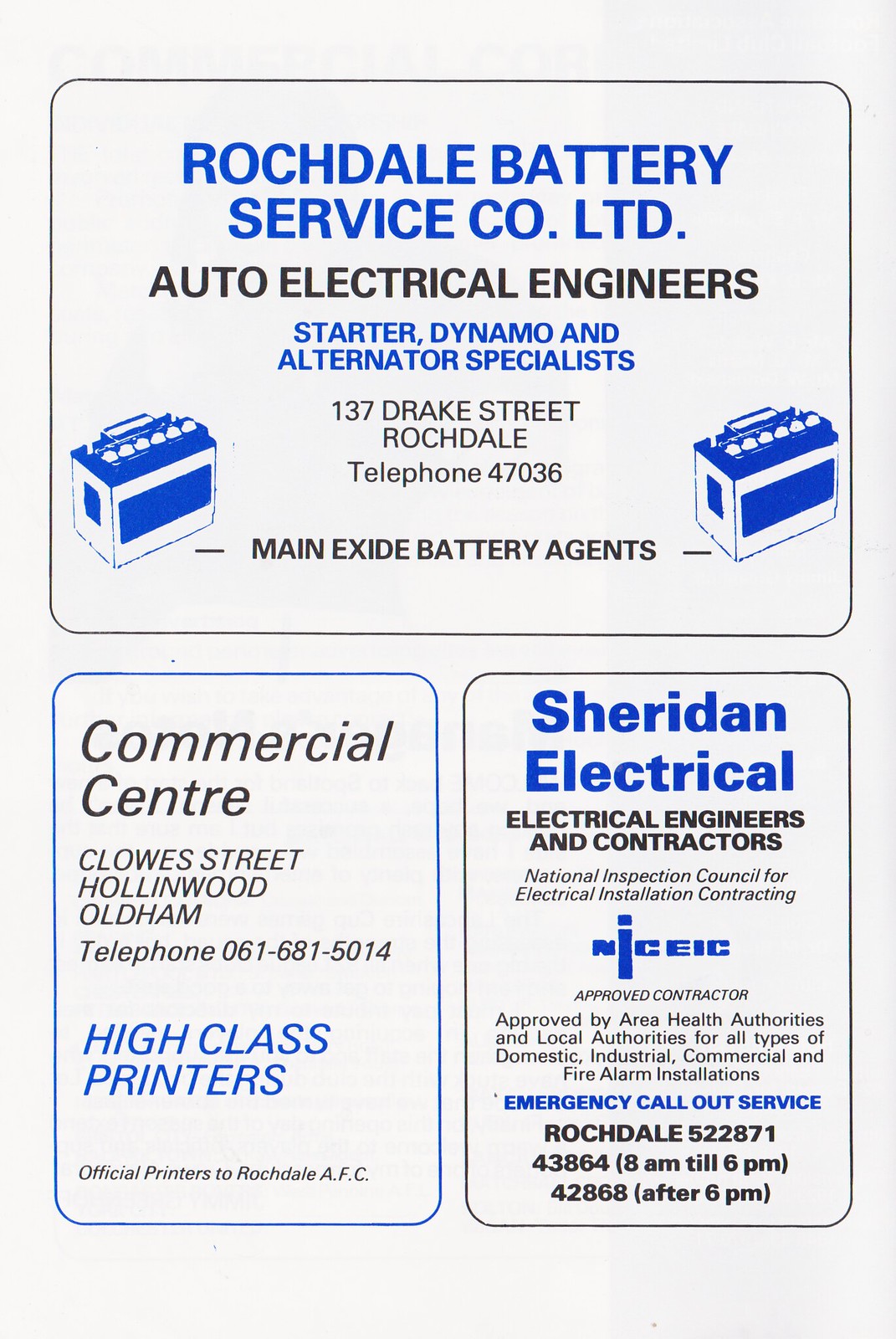This advertisement features a white background with blue and black text, showcasing multiple trades businesses. Dominating the top section is the Rochedale Battery Service Company Limited, highlighted in blue, offering services as Auto Electrical Engineers and specializing in Starter Dynamos and Alternators. Their address is listed as 137 Drake Street, Rochedale, and they are identified as Main Exide Battery Agents. Accompanying this, there is a visual of blue and white batteries to the left.

Below this, in a smaller section to the left, is an ad for Commercial Center, described as High Class Printers. In the bottom right is another ad for Sheridan Electrical, detailing their services as Electrical Engineers and Contractors with Emergency Call Out Service. Additionally, this ad mentions affiliation with the National Inspection Council for Electrical Installation Contracting and includes contact numbers and hours of operation. Together, these ads form a comprehensive promotional sheet for services in the Rochedale area.